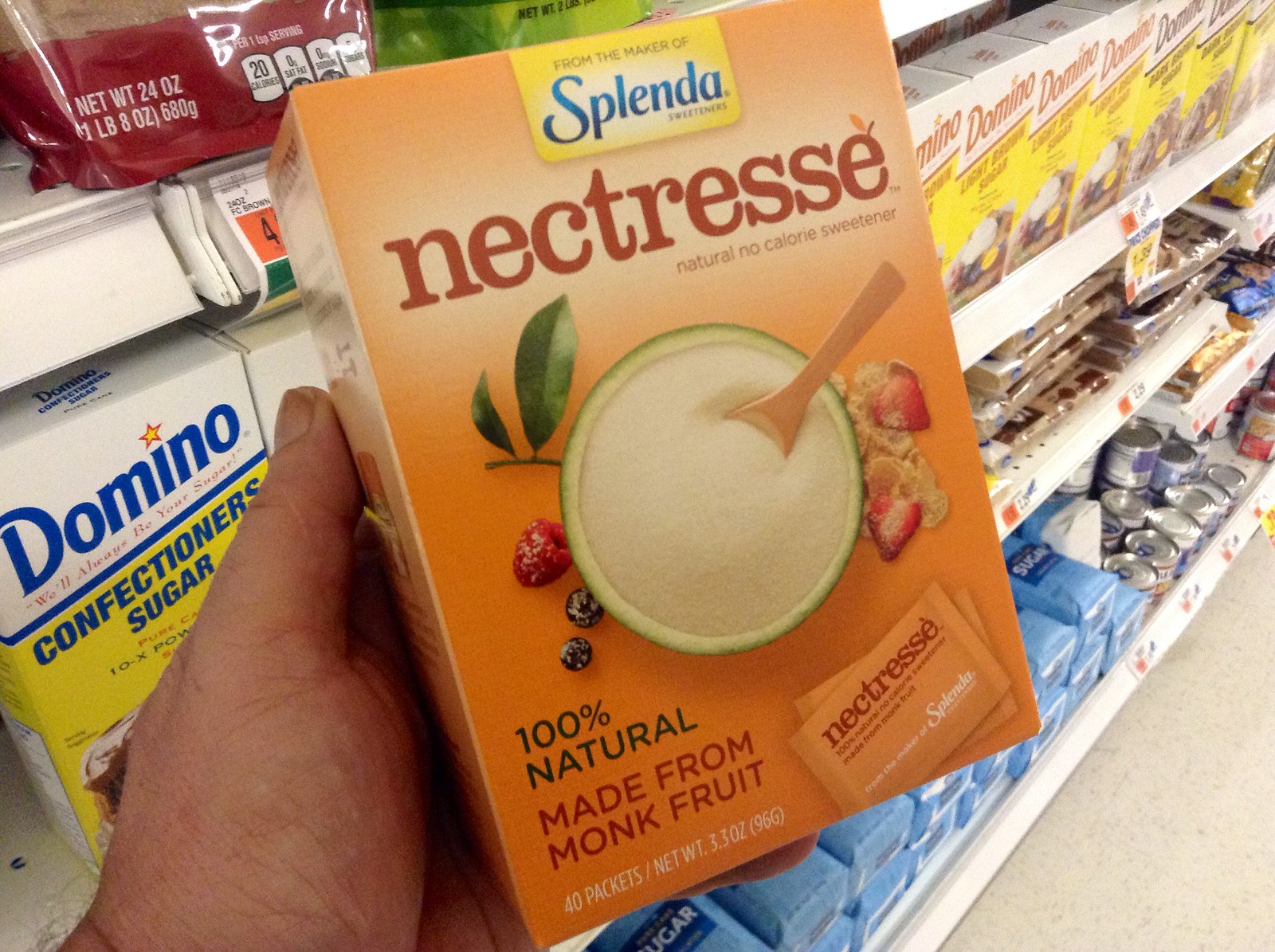In this vibrant photograph taken inside a grocery store, the focus is on the Sweetener Aisle. A hand holds a box of Splenda's Nectresse, featuring a design with a green bowl and a wooden spoon filled with sweetener. Proudly labeled as 100% natural, the product is made from monk fruit and is available in individual packages. The background showcases an array of sweetener options, including neatly stacked boxes of Domino's Confectioners Sugar. On the bottom shelf, large blue 5-pound bags of granulated sugar sit next to cans of condensed sweetened milk. The middle shelf displays clear packages of brown sugar, while the top shelf houses boxes of Domino's Light Brown Sugar, advertised at $1.99 with an accompanying sign. The arrangement and variety encapsulate the diverse sweetening options available to shoppers.